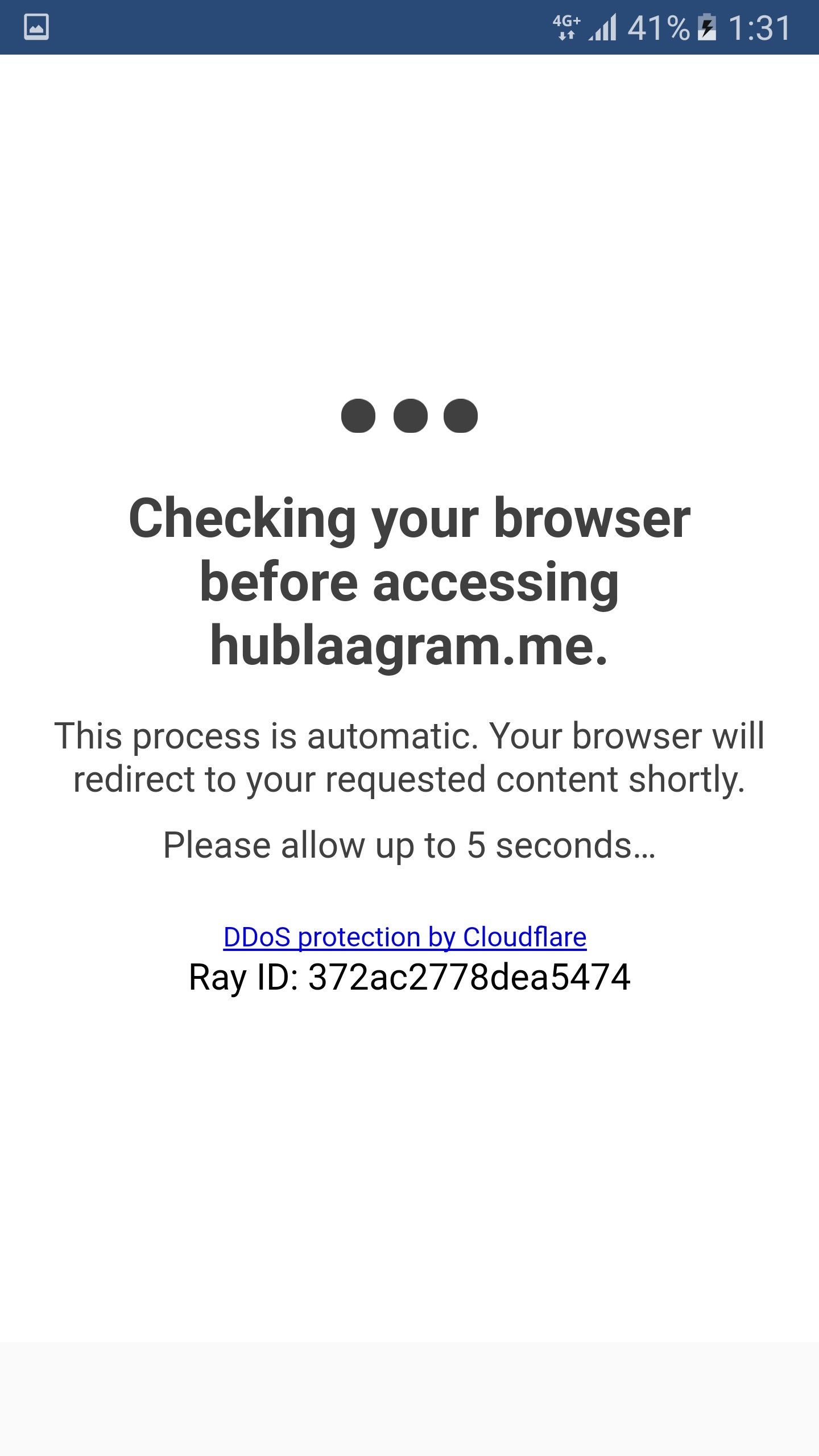A detailed description of the webpage displayed on a smartphone screen:

The image shows a smartphone screen displaying a web page with the title "Checking your browser before accessing this site." This page is typically encountered when trying to access websites that employ advanced security measures like DDoS protection or require specific plugins. The purpose of this page is to ensure the user's device meets necessary security criteria before granting access.

At the top of the screen, there is a blue bar, containing a small image or logo on the left side. In the top right corner of the bar, the phone's status indicators are visible, showing the time (1:31 PM), the charging battery status at 41%, and full 4G network signal bars.

Below the bar, the main content starts with a heading that says "Checking your browser before accessing this site." Just above this heading, there are three large, identical black dots aligned horizontally. These are likely indicating a loading or processing state.

The screen explains that the process is automatic and that the browser will redirect to the requested content shortly. A message underneath advises users to "Please allow up to five..." seconds for the process to complete.

Further down, a notice mentions, "DDoS protection by Cloudflare," highlighted in blue text. Directly beneath this, an "Array ID" is displayed, consisting of a series of numbers and letters, evidencing the unique identification for this specific security check.

The rest of the webpage features a clean, white background, contributing to the overall simplicity and clarity of the message.